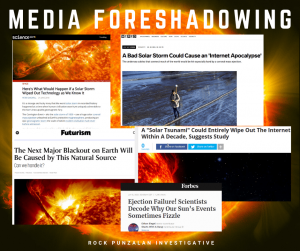The page features a striking composition with a dark, almost black background. Dominating the center is a large, vividly glowing orange sun, surrounded by a yellow outline and flares that radiate outward, giving the impression of it being ablaze. This fiery sun occupies most of the central space, contrasting starkly with the inky sky that frames it.

At the top of the page, the words "MEDIA FORESHADOWING" are emblazoned in bold, white capital letters, making them stand out against the dark background. Encircling the sun is a collage of several headlines, each suggesting foreboding implications of solar activity. 

One prominent headline reads, "A BAD SOLAR STORM COULD CAUSE AN INTERNET APOCALYPSE," accompanied by an image of a man looking down at his phone, set against a bluish-gray backdrop. Below this, another headline warns, "A SOLAR TSUNAMI COULD ENTIRELY WIPE OUT THE INTERNET WITHIN A DECADE, SUGGESTS STUDY." The final headline included in the collage states, "EJECTION FAILURE, SCIENTISTS DECODE WHY OUR SUN'S EVENTS SOMETIMES FIZZLE."

At the very bottom of the page, the phrase "Rock Ponslum Investigative" is displayed, hinting at the source or nature of the compilation. The overall design of the page crafts a vivid scene of impending doom posed by solar phenomena, effectively highlighted by the dramatic imagery and stark headlines.